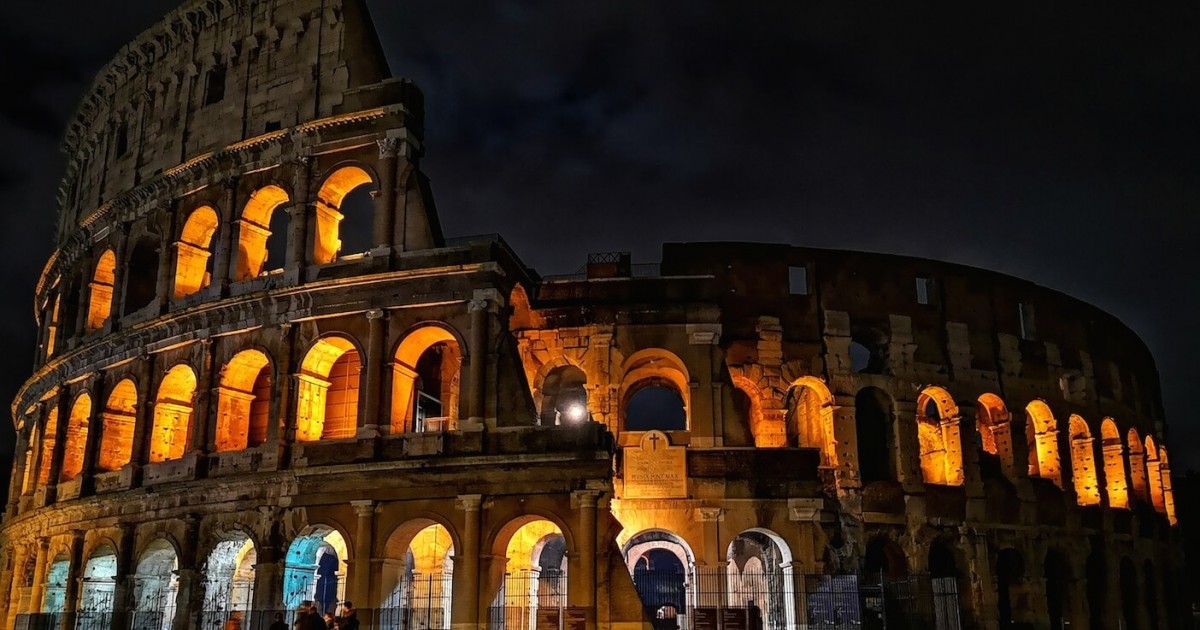The image depicts the Colosseum in Rome, Italy, illuminated dramatically against a dark night sky. The ancient stone structure, renowned for its historical significance as a sports arena, takes on a mesmerizing appearance with glowing orange and golden lights accentuating its arches and multiple levels. The left side of the Colosseum remains intact, showing all three stories and the top, while the right side is partially collapsed. The brightly lit archways allow glimpses of the glowing interior, contrasting vividly with the deep black sky. A black-colored wall or fence can be seen at the bottom of the image, adding to the scene's overall depth and framing the view of this iconic monument.